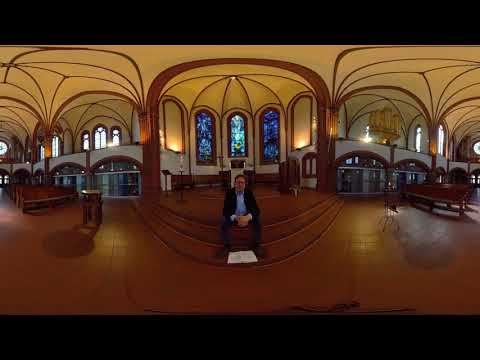This indoor photograph captures the tranquil interior of a church, with a man as its focal point. He sits pensively at the top of a low, wide wooden staircase at the front of the sanctuary. The man, dressed in a blue long-sleeved shirt, a dark jacket, and dark pants, has dark hair and is staring intently at the camera. An open white book lies on the step below him. Surrounding him are old-fashioned wooden pews that frame both sides of the image, creating an aisle leading up to the stairs. The floor is a rich dark brown wood, complementing the church's extensive wood detailing. The ceiling is primarily off-white with elegant dark wood accents intersecting it. Prominently displayed behind the man are arched stained glass windows, adding a touch of color and sacred ambiance to the serene scene. A balcony space is visible above, enhancing the room’s architectural depth and character.